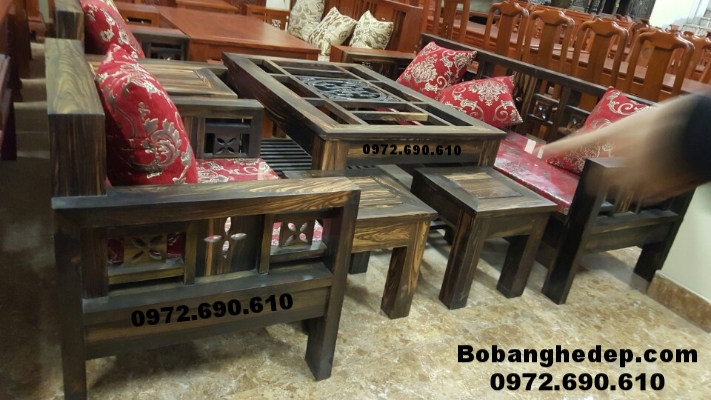This image depicts an indoor setting, likely a furniture store, showcasing an array of wooden furniture in a tightly crammed arrangement. Dominating the photograph are a variety of tables and chairs in different shades of brown, from dark to light. The furniture presents a Southeastern aesthetic. In the background, there are several reddish-brown tables and chairs, some adorned with white pillows featuring light brown embroidery. Centered and foreground in the image is darker brown wooden furniture, including a bench with a red seat and small tables with red and gold embroidered cushions. The most prominent text, repeated across various spots including the bottom right, reads "bobanghedep.com 0972.690.610." This text is also seen on several other pieces within the image.